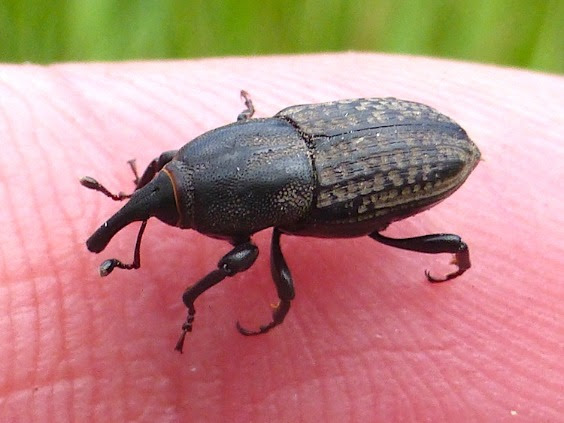The photograph captures a detailed, zoomed-in view of a round, nut-shaped beetle perched on someone's fingertip. The beetle has an oval body with thick black legs that end in rounded hooks, three on each side. Its head, featuring two black antennae and a downward-curving horn or large nose, is directed towards the left of the frame, while its bottom points to the right. The beetle's back is predominantly black with various grey and brown pits. The background of the image is fuzzy and green, suggesting it could be grass, indicating the photograph was likely taken outdoors in daylight. The clarity of the image allows for a clear view of the ridges on the person's fingertip, further emphasizing the beetle’s detailed features.